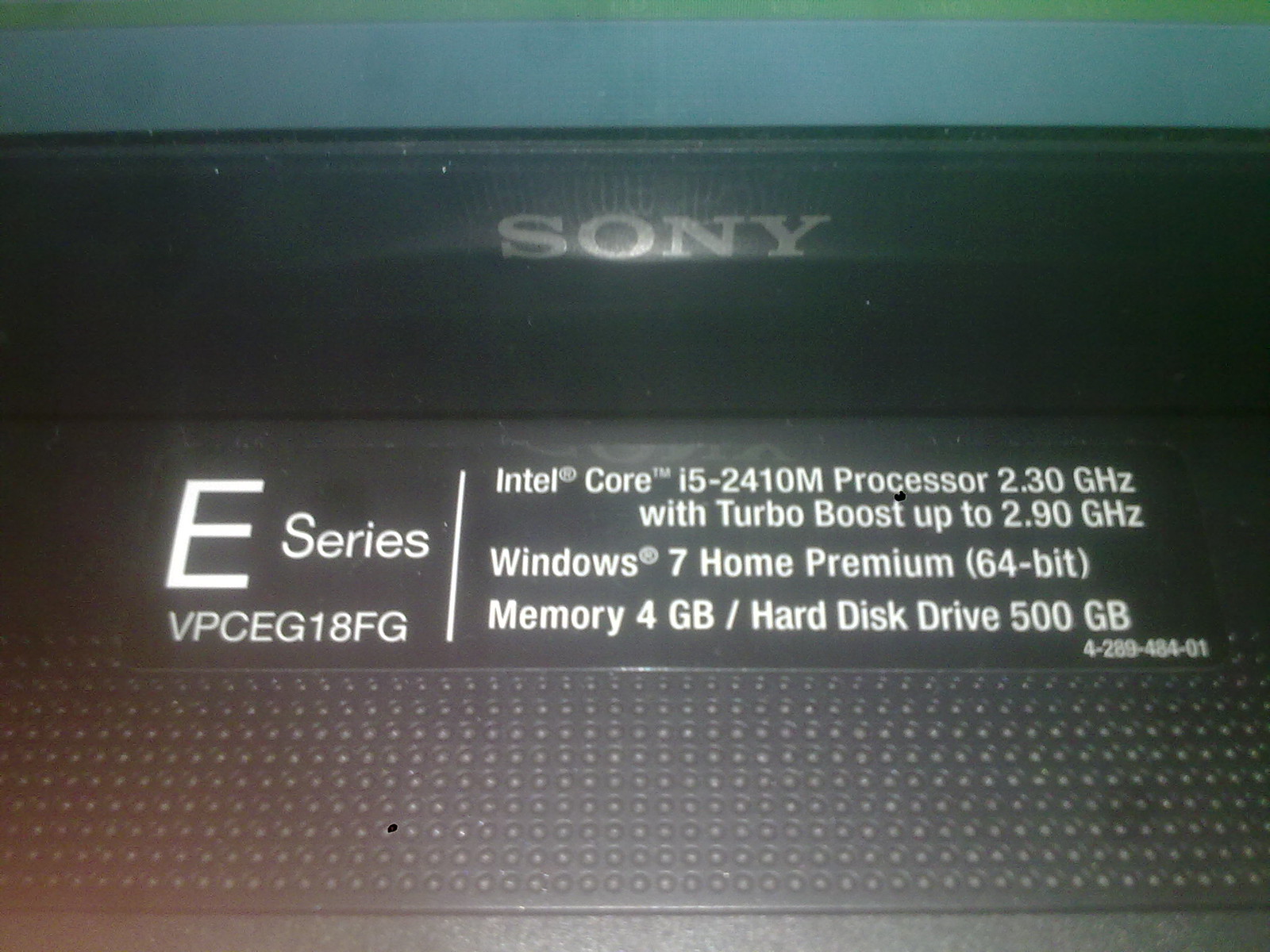This detailed, composite caption is based on the shared and repeated information from the three descriptions:

The image showcases a close-up of an information card from a black, box-like electronic device, identified as a laptop by Sony. The prominent silver "SONY" logo is visible at the top, behind a clear acrylic cover. Below the logo, the label is a black rectangle with white font, reading from left to right: "E-Series VPCEG18FG," with a white line underneath it separating the model number from the specifications. The right side of the label details the device's features: "Intel Core i5-2410M Processor 2.30GHz with Turbo Boost up to 2.9GHz, Windows 7 Home Premium 64-bit, Memory 4GB, Hard Drive 500GB, 428948401." The image's overall visual composition includes elements of black, white, and slight accents of light blue and green at the top, suggestive of the display area, with the hard drive taking up the bottom half of the image.